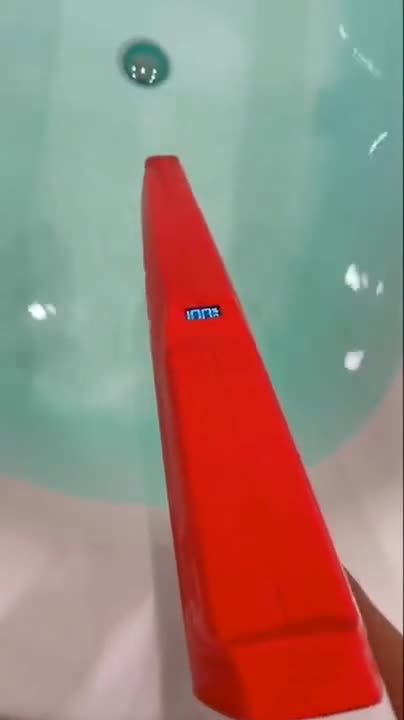The image depicts a peculiar scene featuring a red, elongated device that extends from the bottom right corner of the frame and rises towards the center top of the vertically-oriented rectangular background. The object, which narrows slightly towards its tip, begins with a white base before transitioning into red. It features a small digital screen displaying the number 100, hinting at its potential function but leaving its exact purpose ambiguous. The frame's majority is filled with a mint green or lime green water-like substance, suggesting the setting might be a sink, bathtub, or pool. The device, appearing almost as a vacuum or specialized tool, is partially submerged, adding to the mystery of its function—whether it's measuring, filtering, or aerating the water remains uncertain. Against the blurry gray and light purple backdrop, this enigmatic object stands out, inviting curiosity and speculation.